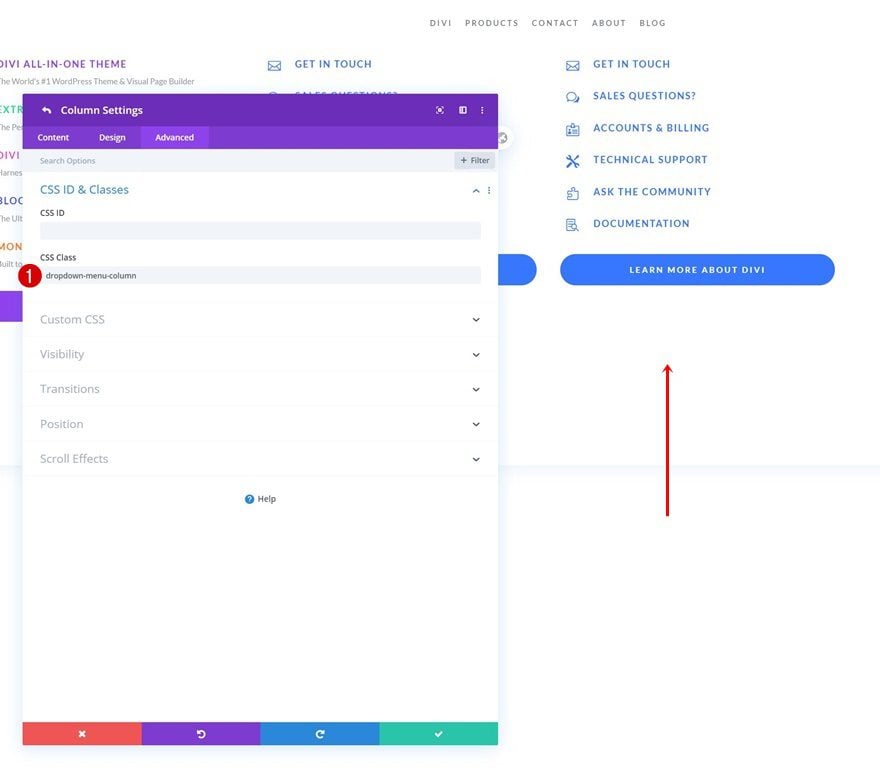This image depicts a web page focusing on a pop-up box with a purple header labeled "Column Settings" accompanied by an adjacent back button. Below this header, the pop-up box offers three main categories: Content, Design, and Advanced. Directly beneath these options is a gray search bar titled "Search Options." 

The first visible field under "Search Options" is labeled "CSS ID" and features an empty text box intended for user input. Following this, there is another field labeled "CSS Class" with a pre-filled text box containing the term "dropdown-menu-column."

Further down, the pop-up box expands into various dropdown sections including "Custom CSS," "Visibility," "Transitions," "Position," and "Scroll Effects." Each section is likely intended to provide additional customization settings for the web page column.

At the bottom right corner of the pop-up box, there is a question mark icon, presumably serving as a help button for user assistance.